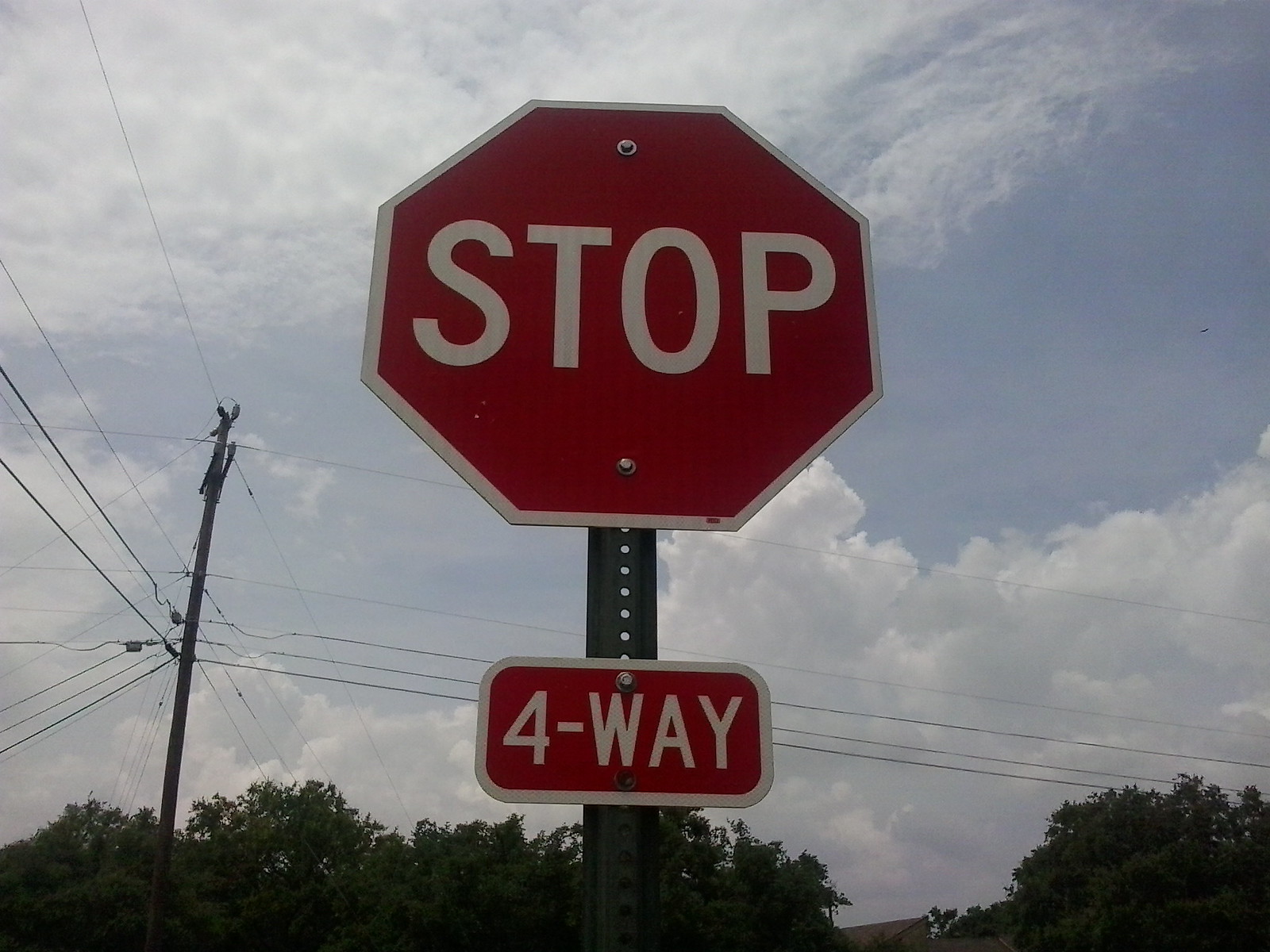The photograph captures a typical red and white stop sign prominently centered, dominating much of the frame. The stop sign is octagonal, displaying the word "STOP" in bold, white block letters against the red backdrop. Directly beneath it, a smaller sign indicates "4-WAY," also in white letters on a red background, signifying a four-way stop intersection. In the background, the sky is a clear blue adorned with several fluffy, white clouds. Power lines stretch horizontally and vertically across the scene, intersecting behind the stop sign. At the bottom edge of the photo, the tops of trees peek into the frame, adding a touch of greenery.